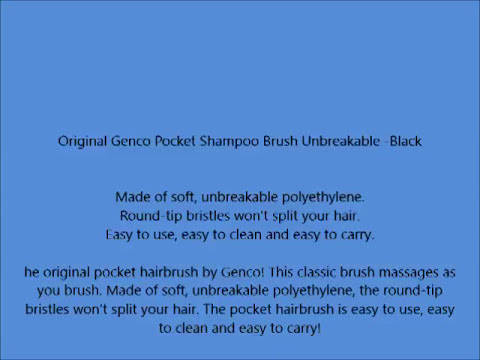The image features a medium blue background with centered black text promoting the "Original Genco Pocket Shampoo Brush." The text reads: "Original Genco Pocket Shampoo Brush, Unbreakable, Black." Below, it details, "Made of soft, unbreakable polyethylene. Round tip bristles won't split your hair. Easy to use, easy to clean, easy to carry." Further down, the text repeats with slight variations: "The original pocket hairbrush by Genco! This classic brush massages as you brush. Made of soft, unbreakable polyethylene. The round tip bristles won't split your hair. The pocket hairbrush is easy to use, easy to clean, and easy to carry!" This structured advertisement emphasizes the brush's durability, gentle bristles, and user-friendly design, all set against a medium blue backdrop.